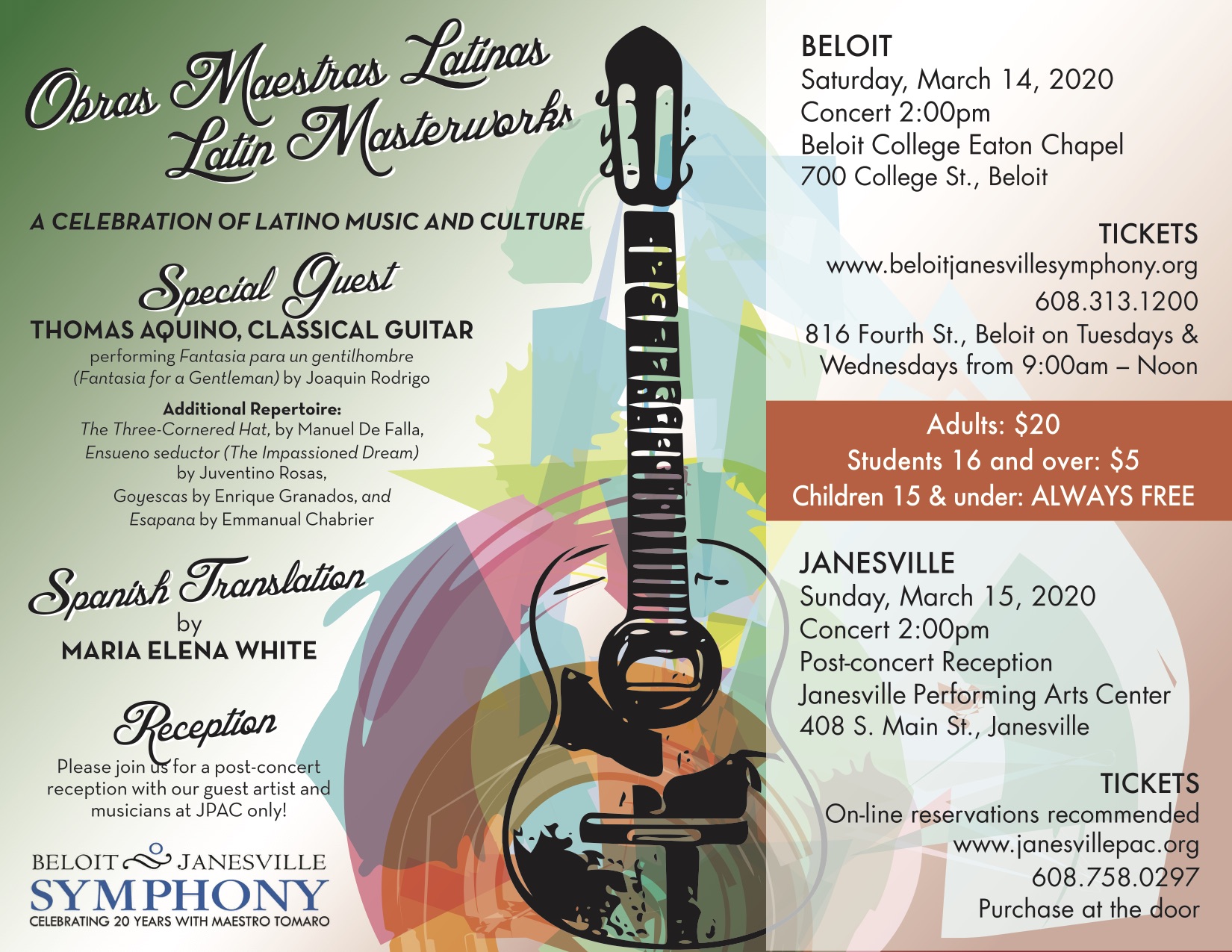This is a detailed promotional poster for the Beloit Janesville Symphony Orchestra's celebration of Latino music and culture. The centerpiece of the design is a black artistic illustration of a classical guitar, accentuated by light, colorful patterns in shades of pink, green, and blue. The background transitions from a greenish gradient to a reddish one, giving it a dynamic look. 

At the top left corner, the poster features the title "Opras Maestras Latinas" followed by its English translation, "Latin Masterworks," in black and white text. It's a celebration of Latino music and culture, featuring special guest Thomas Aquino on classical guitar performing "Fantasia para un Gentilhombre" ("Fantasia for a Gentleman") by Joaquin Rodrigo. The additional repertoire includes "The Three-Cornered Hat," with a Spanish translation by Maria Elena White. 

Important event details are provided on the left side, such as a post-concert reception with the guest artists and musicians exclusively at J-PAC. On the right side, specific event information is included: 

- Date & Time: Saturday, March 14th, 2020 at 2:00 p.m.
- Venue: Beloit College Eaton Chapel, 700 College Street, Beloit.
- Ticket Information: Adults $20, students (16 and over) $5, children (15 and under) free.
- Contact Details: Includes address, website information, and phone number with ticket office hours (Tuesdays and Wednesdays from 9 to noon).

The text at the very bottom left notes "BELOIT JANESVILLE SYMPHONY" in blue capital letters, with another line in black capital letters stating "Celebrating 20 years with Maestro Tomorrow." Overall, the poster is densely packed with comprehensive information about the event, making it clear and convenient for all potential attendees.